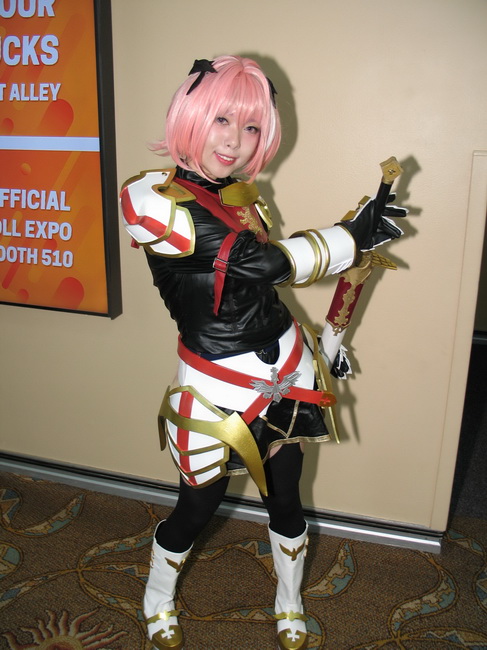The image captures an Asian woman fully immersed in cosplay, likely at a comic-con or similar expo. She sports a shoulder-length light pink bob wig, adorned with small black bows. Her costume is a detailed ensemble consisting of black pants, a black top with white body armor accented by gold and red straps, a white skirt with red trim, and white boots decorated with gold markings. Black gloves with white accents complete her look. She confidently poses for the camera, her head slightly tilted and a smile on her face. She holds a sword, with the blade partly sheathed, contributing to her fierce yet composed demeanor. The background features a light beige wall casting a shadow, indicative of the lighting. To her left, a partially visible black-framed sign reads fragmented text: "CKS... Alley... OFFICIAL... Expo... 510," suggesting the setting is an official expo or convention. The floor beneath her is a brown carpet with blue and tan floral patterns.